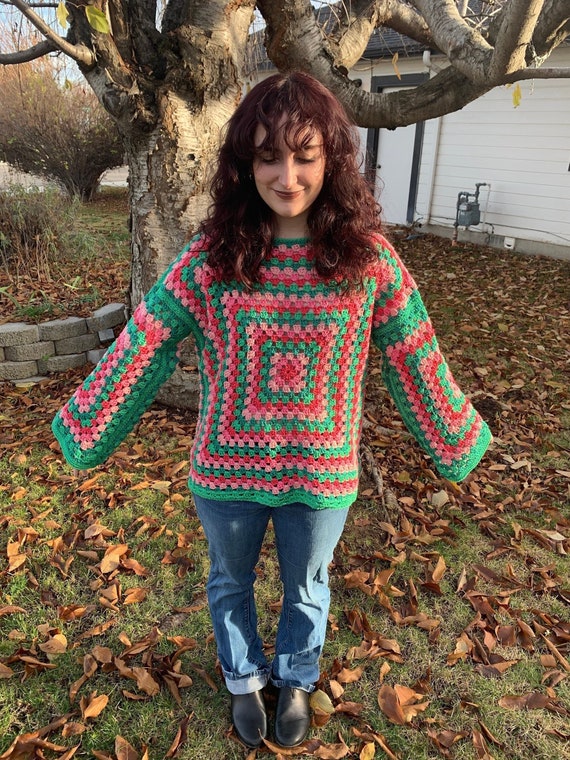In this photograph, a young woman is posing outdoors in a yard filled with fallen leaves, giving a sense of autumn. She is wearing a colorful crocheted sweater in the granny square pattern, featuring dark pink, light pink, green, and blue squares, paired with blue jeans and black shoes. Her arms are angled slightly away from her body as if to show off the sleeves and intricate design of her sweater. She stands with her feet together, her head bowed slightly, eyes closed, and a soft smile on her face. Her long, reddish-brown curly hair, highlighted beautifully by the sunlight, frames her face with longer curly bangs. In the background, a thick, leafless tree with large branches dominates the scene. To the left of the tree, a garden area bordered by gray cinder blocks is visible. On the right, the wood siding of a house is partially seen, along with a silver gas meter attached to the building. These elements, combined, create a serene and detailed autumnal portrait.